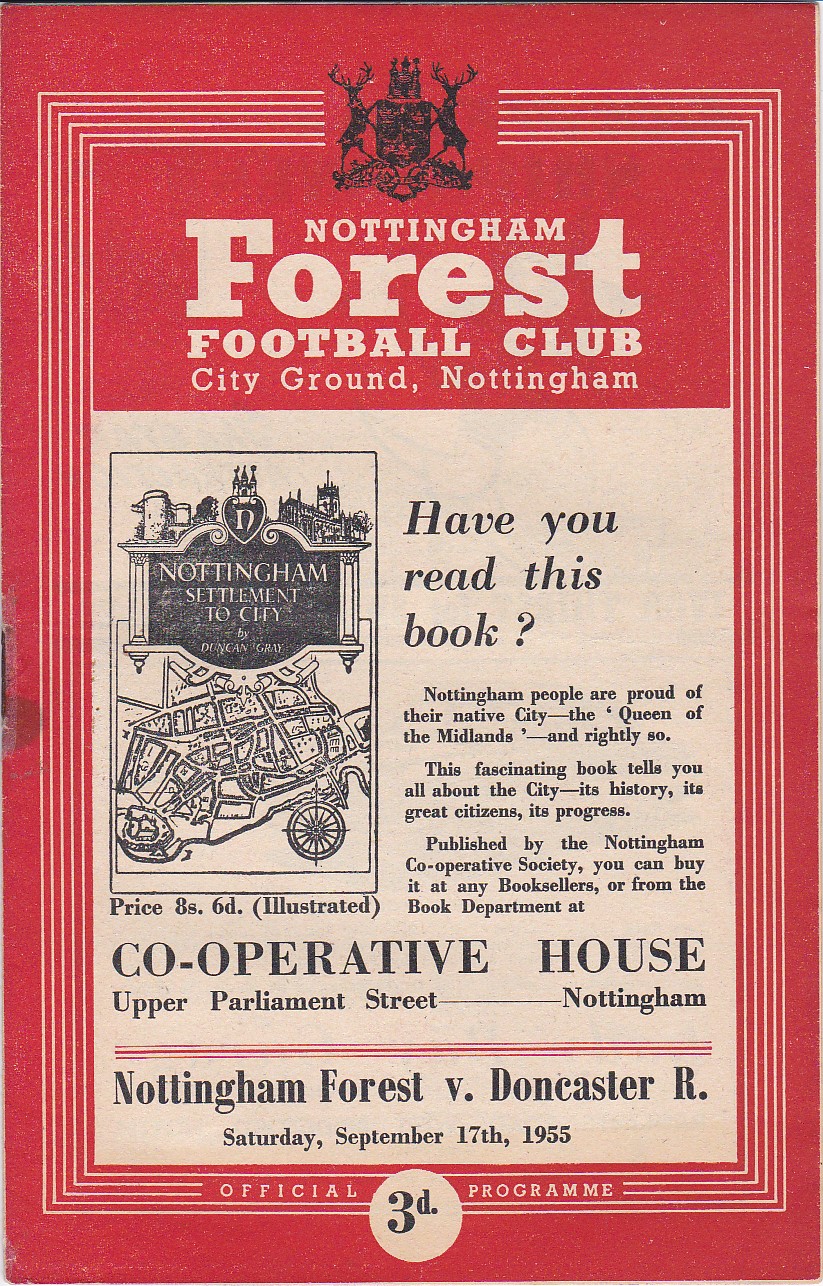The image is a vintage poster for the Nottingham Forest Football Club, prominently featuring a solid red background with light beige stripes forming a border around the central text. At the top center, a crest symbol flanked by deer stands out, followed by bold white text that reads "Nottingham Forest Football Club" and "City Ground, Nottingham." Below this, the central area contains a large block of white with intricate black text highlighting an intriguing book about Nottingham. The text reads: "Have you read this book? Nottingham people are proud of their native city, the Queen of the Midlands, and rightly so. This fascinating book tells you all about the city, its history, its great citizens, its progress. Published by the Nottingham Cooperative Society. You can buy it at any booksellers or from the book department at Cooperative House, Upper Parliament Street, in Nottingham." To the left of this text, a symbol and a map of Nottingham, titled "Nottingham Settlement to City by Duncan Gray," are displayed. Further down, it lists "Nottingham Forest vs. Doncaster Rovers, Saturday, September 17th, 1955," and the bottom ends with "Official Programme 3D" within a white-lined border.